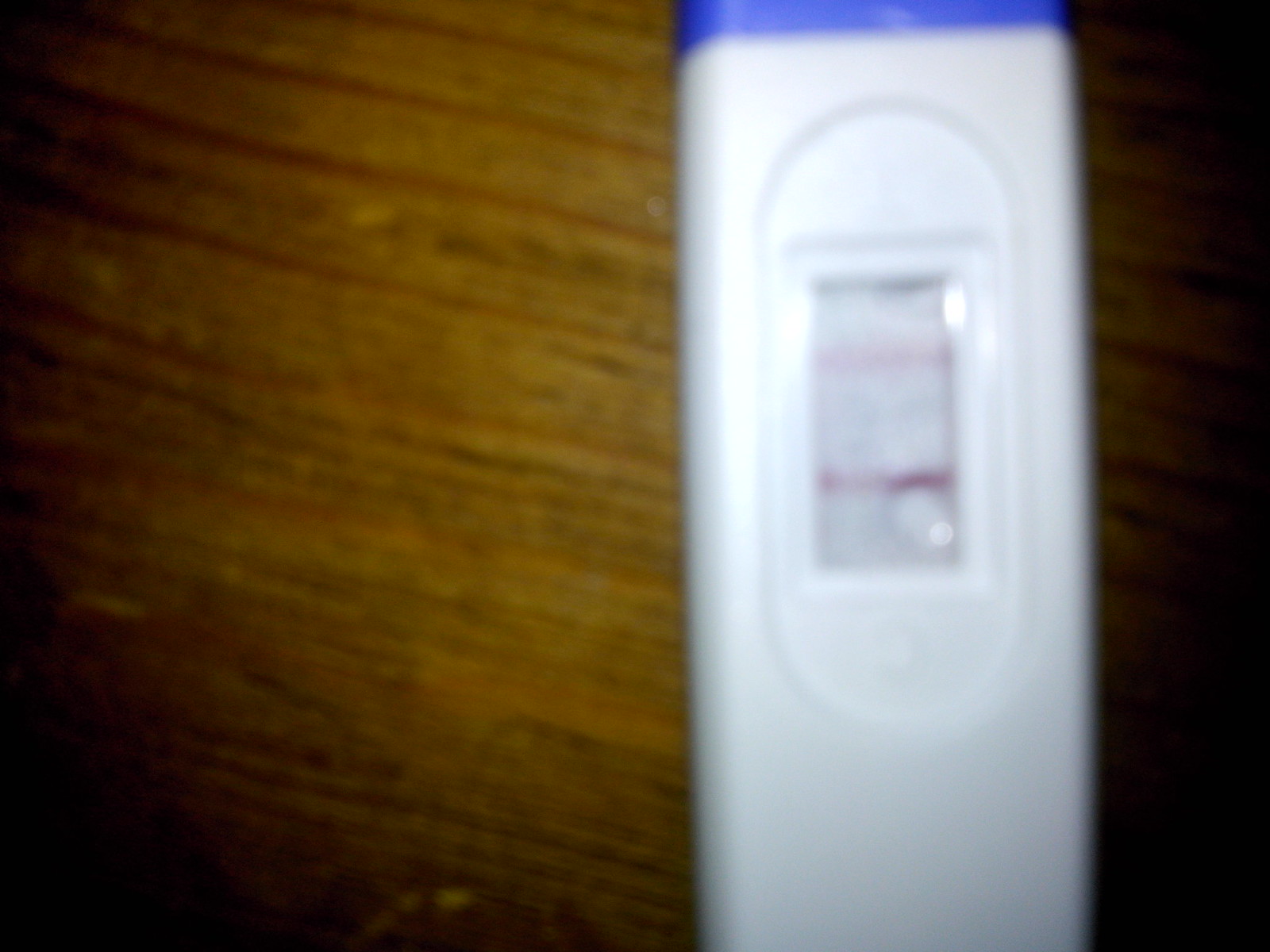This photograph depicts an ovulation test placed vertically on a surface with a walnut grain pattern, likely a faux wood finish in a medium to dark brown hue. The test device has a white body with a bright royal blue trim at the top. The readout section is rectangular and situated near the top of the device. Due to the extreme blurriness of the image, the details of the test result are difficult to discern clearly. However, a darker line is visible, along with a fainter, lighter line towards the top of the readout window. The distinct design and color scheme of the test are indicative of a well-known brand.